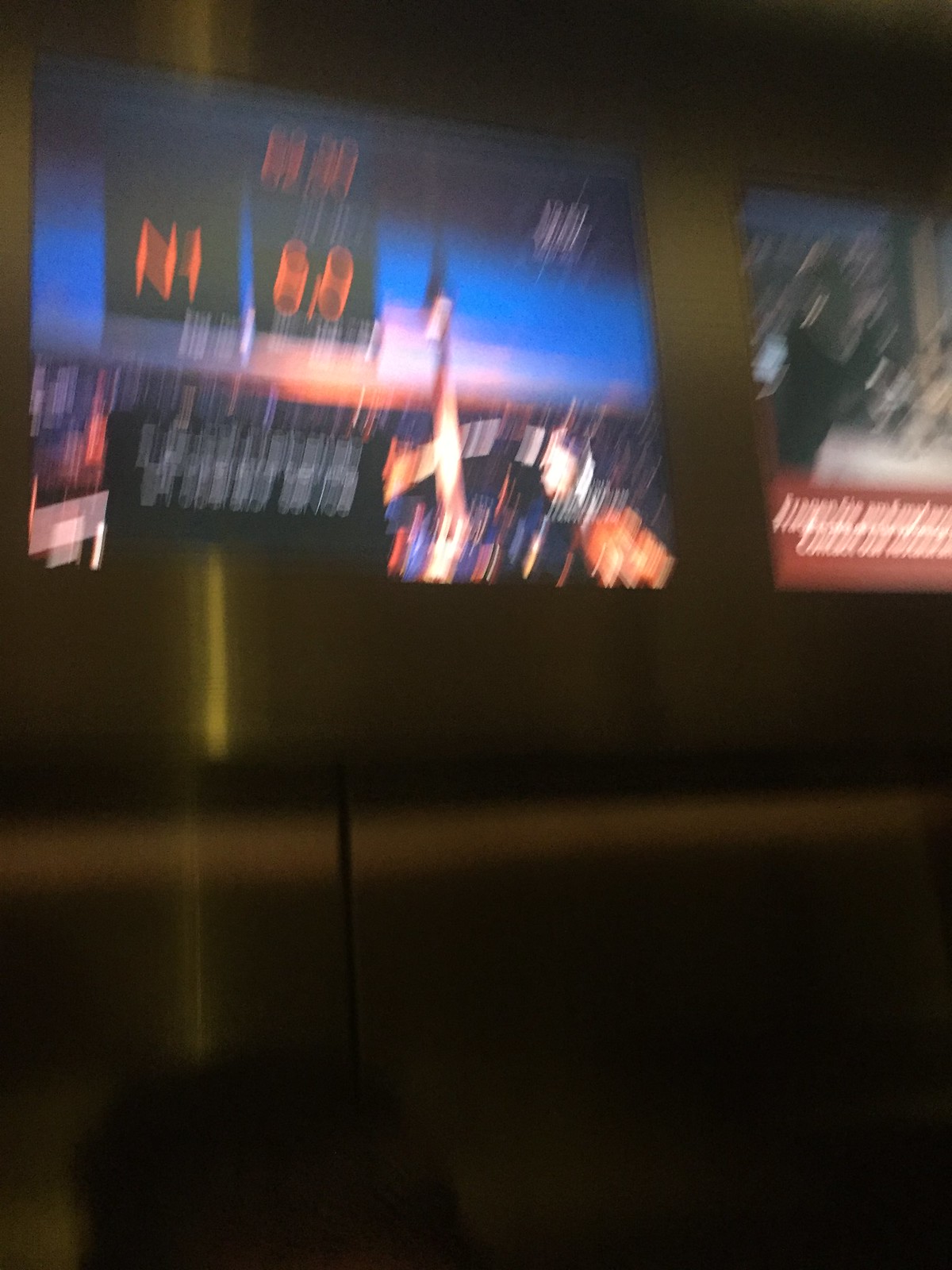This night-time photograph captures a scene filled with motion blur, adding a dynamic and somewhat chaotic effect to the image. The lower half of the frame is predominantly dark, suggesting the absence of ambient light or objects in that portion. A faint, light-grey horizontal line runs across the image, possibly indicating a barrier or reflective surface. The upper half showcases two illuminated billboards positioned against the night sky. 

On the right-hand side, an extremely blurred billboard features a segment with red and white text, though its details are indistinguishable. To the left, a slightly clearer billboard displays what seems to be a distant cityscape at night. The city lights twinkle beneath a gradient sky transitioning from the hues of sunset into deep blue. Additionally, there are two smaller digital displays embedded in the scene, one displaying a letter and the other numbers in an unclear orange font. The amalgamation of blurred motion and illuminated billboards against the darkened lower half creates an abstract, almost surreal night-time cityscape.